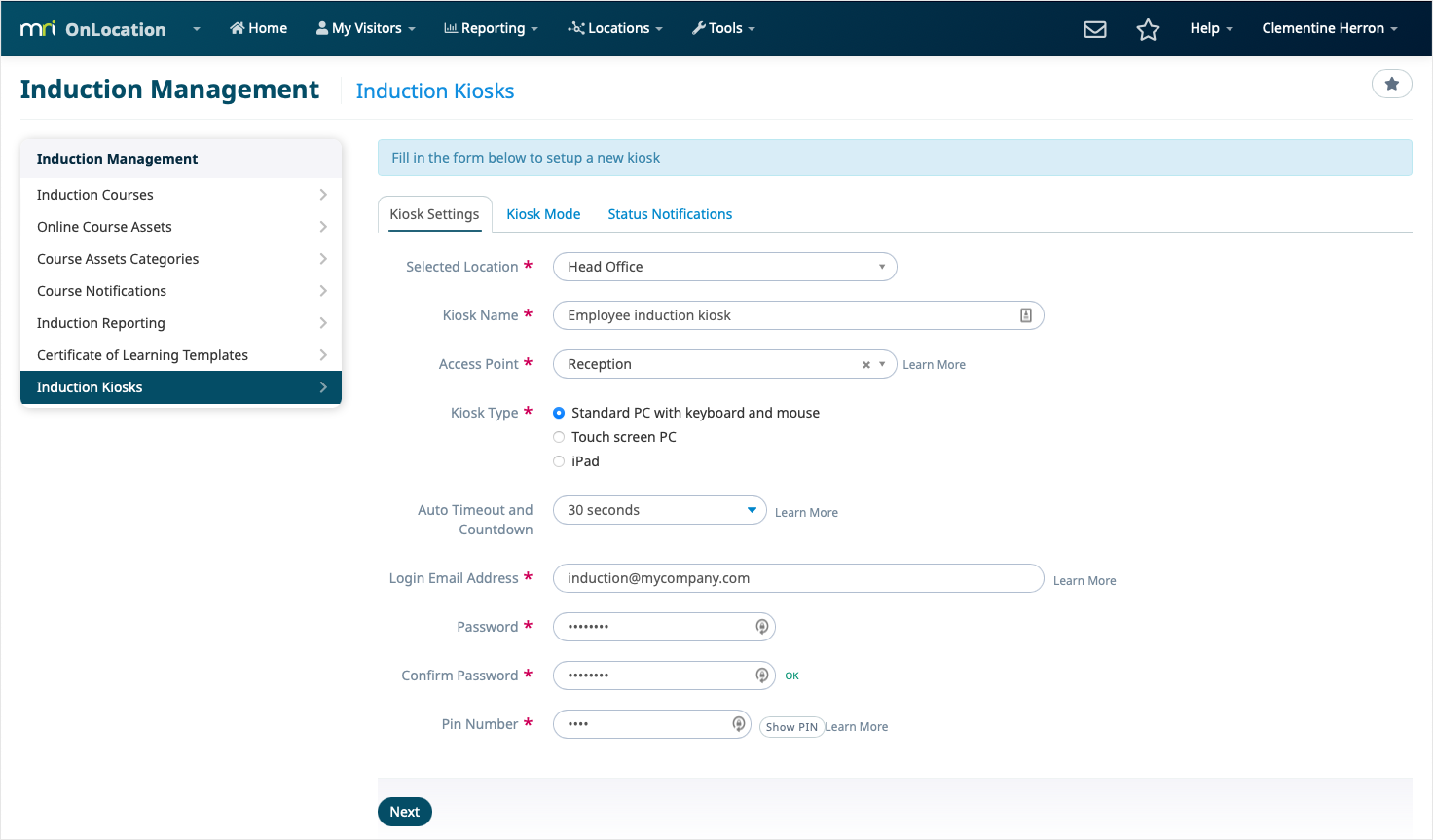This is a detailed caption for a screenshot of a web console, designed for the management and configuration of induction kiosks:

---

The screenshot captures a web interface titled "Induction Management and Induction Kiosks." At the top of the interface, there’s a black menu bar displaying various options: "MRI on Location - Home," "My Visitors," "Reporting," "Locations," "Tools," and "Options." To the right, there are icons for an email envelope, a star (presumably for bookmarking the page), a help dropdown menu, and the name "Clementine Heron" with a dropdown, suggesting that she is the current logged-in user with an option to log out.

Immediately below the menu bar, in bold text, are the titles "Induction Management" and "Induction Kiosks." On the left side of the interface, there's a vertical menu listing various categories: "Induction Management," "Induction Courses," "Online Course Assets," "Course Assets Categories," "Course Notifications," "Induction Reporting," "Certificate of Learning Templates," and "Induction Kiosks." Each category has caret symbols, indicating expandable sub-menus. The "Induction Kiosks" category is currently selected.

The main section to the right of the vertical menu displays a form for setting up a new kiosk. Prominently titled "Fill in the form below to set up a new kiosk," the form includes three tabs: "Kiosk Settings," "Kiosk Mode," and "Status Notifications." The form fields allow users to specify various details:

- **Selected Location:** Currently set to "Head Office."
- **Kiosk Name:** Labeled as "Employee Induction Kiosk."
- **Access Points:** Set to "Reception."
- **Kiosk Type:** Options include "Standard PC with Keyboard," "Touch Screen PC," or "iPad."
- **Auto Timeout:** Configurable with the current setting at "30 seconds."
- **Login Email Address:** Allows for email input.
- **Password:** With fields for confirming the password.
- **Pin Number:** An additional security feature.

At the bottom of the form, there’s a "Next" button to proceed with configuring further options for the kiosk setup.

---

This richly detailed caption helps to convey the comprehensive functionality available within the web console dedicated to managing induction kiosks.